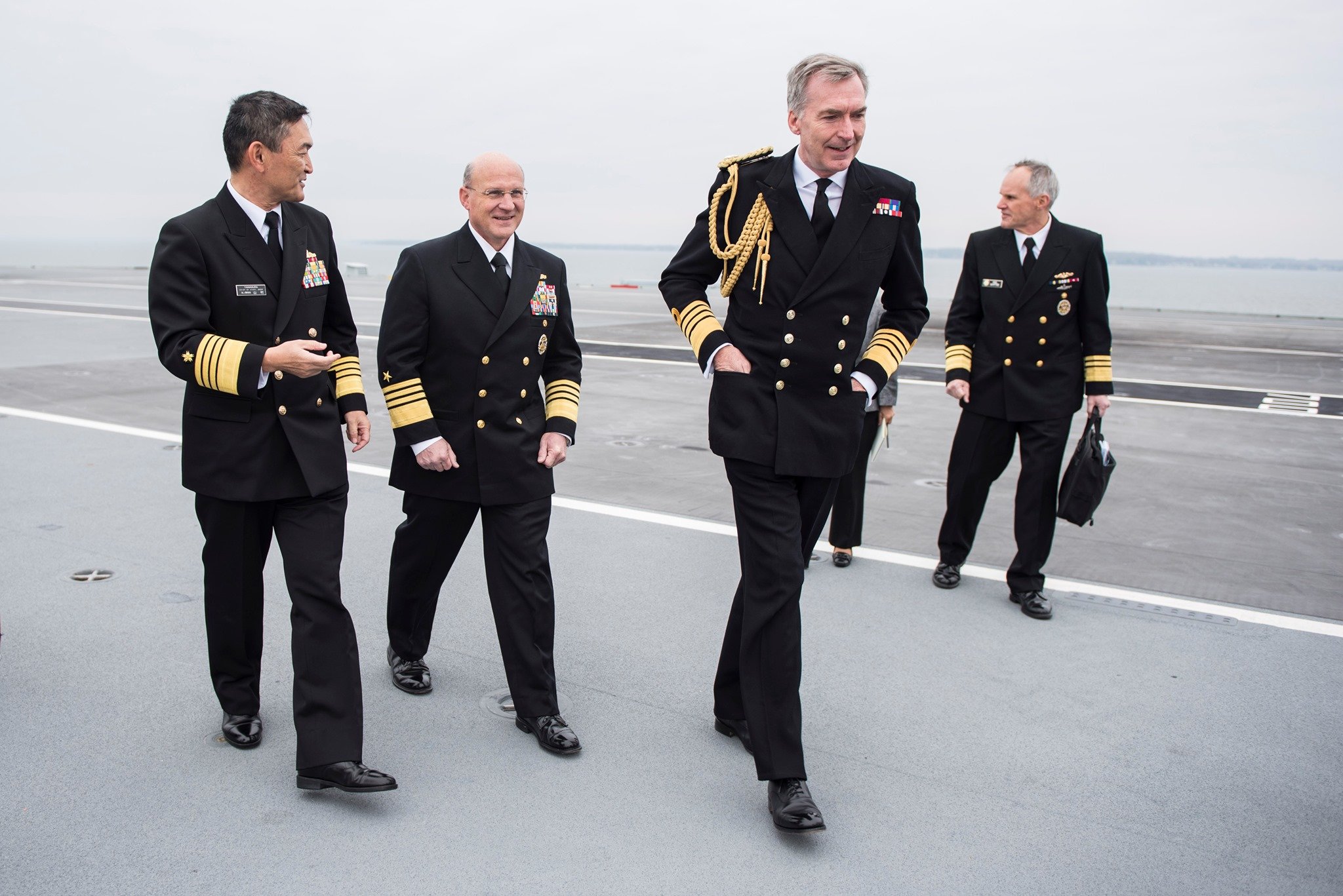The photograph features a group of four high-ranking U.S. naval officers, distinguished by their formal uniforms and the various decorations they wear. They are standing on what appears to be an aircraft carrier, with a gray sky and water visible in the background. Their attire includes black double-buttoned blazers adorned with gold buttons and gold stripes on the sleeves, signifying their rank. Each officer sports a chest full of medals and colorful badges, indicating their decorated service history. 

On the far left is an officer with dark hair, possibly of Asian descent, who is smiling and engaged in conversation. He is followed by a bald-headed officer with a fringe of hair around his head, also fully decorated with medals. The third officer has a slightly fewer number of medals and features a distinctive golden braid on his right shoulder, often associated with distinguished roles or honorific titles. The last officer, partially obscured, boasts a notable large medal below his ribbon bar and carries a satchel. A woman, partially hidden behind the group, seems to be a part of the assembly, adding to the total count of five people. Bright expressions and a sense of camaraderie suggest that they are enjoying their interaction and whatever event they are partaking in.